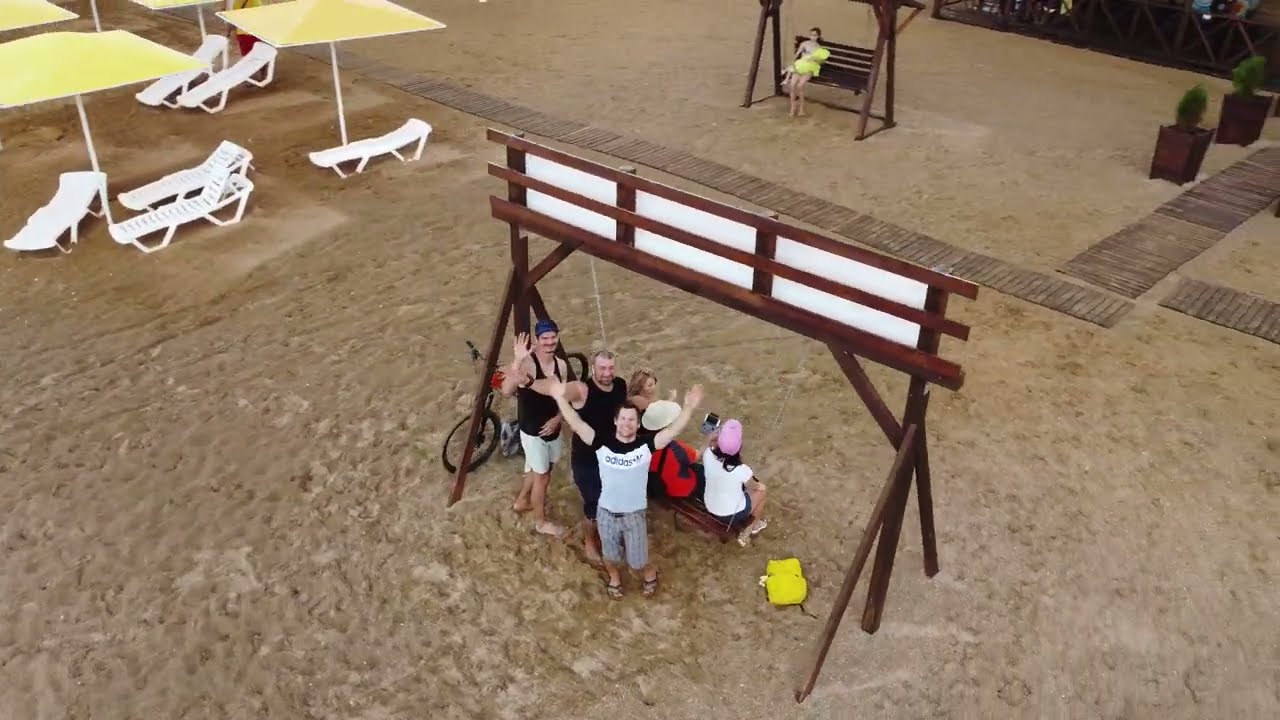In this bright daytime image, set against a backdrop that suggests a beach or a park adjacent to a hotel, we see a central wooden swing structure with several people positioned around it. Predominantly marked by tan sand and a wooden walkway that splits to the left and right, the scene includes multiple beach elements. On the left side of the image, white lounge chairs are arranged under yellow parasols. In the middle, beneath the wooden swing structure, three men command attention: one in a bluish t-shirt with his arms raised in a victory pose, another in a black tank top also waving, and a third in black attire giving a friendly wave. A pink capped individual kneels nearby, and a white-hatted person is also seen kneeling. A woman holding a child sits on another swing in the background near the center, with a stationary bike leaning against the swing posts. The image captures a moment of leisure and camaraderie, reflected in the smiling, waving individuals who are the focus of the photograph. The colors predominantly featured are tan, white, brown, yellow, pink, red, black, and green, accentuated by green potted plants that line sections of the walkway.